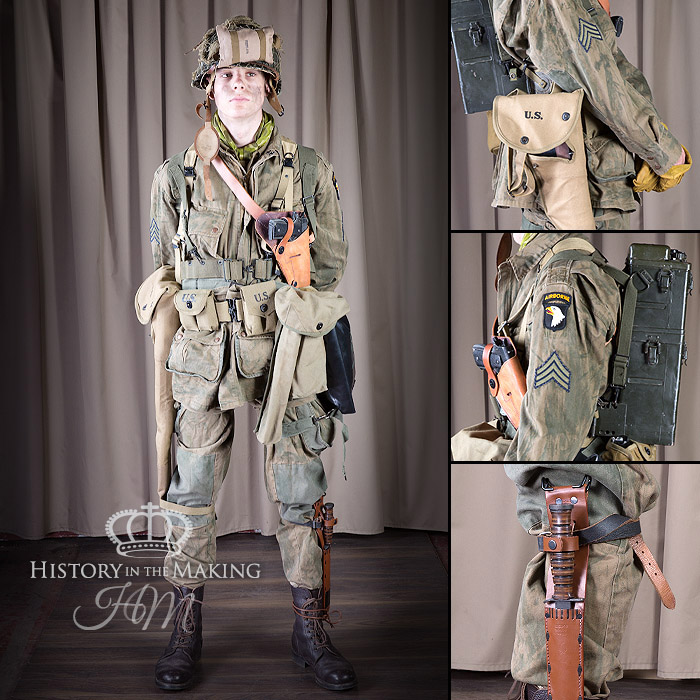This detailed image illustrates a U.S. military soldier, potentially an Airborne officer, showcased in four distinct frames. On the left, we see a full-body view of the soldier standing with hands behind their back, clad in a brown U.S. military uniform highlighted by green accents and various compartments. The soldier sports a brown helmet with a small pillow-like item at the front and a green inner clothing layer. A camouflage scarf is draped around their neck, and the chinstrap of the helmet hangs loosely. Tactical gear adorns their uniform, including a gun strapped to their chest and a knife secured in a protective case on their ankle. Black army boots complete their attire. The soldier's waist features a pouch labeled "U.S." and they carry a backpack. To the right, three stacked frames offer zoomed-in views: the first focuses on the soldier's right shoulder down to their black combat boots, the second provides a clear view of the backpack and left shoulder, and the third spotlights the knife on the left ankle. The bottom left of the larger frame is marked with the insignia "History in the Making."